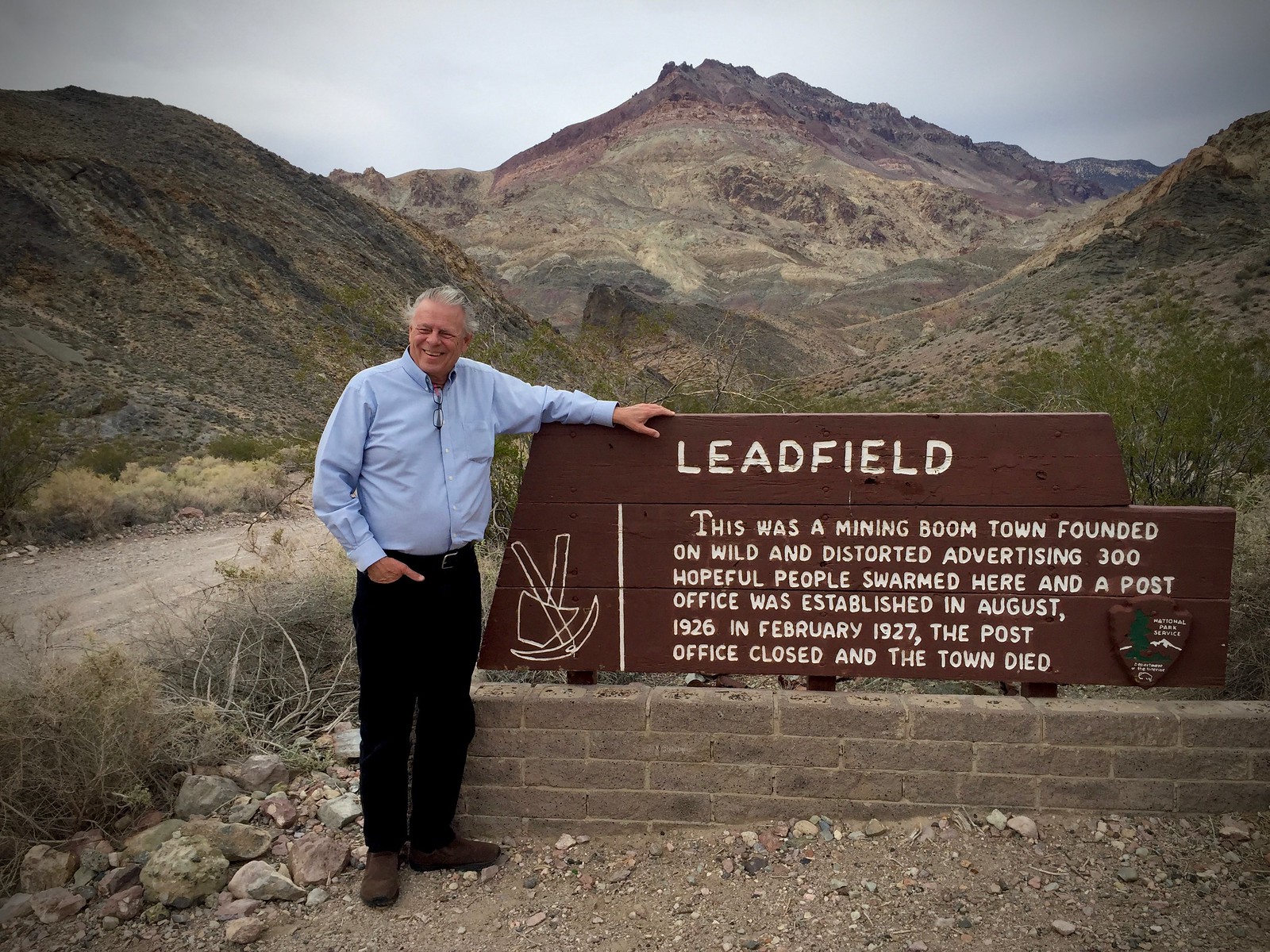This detailed image captures an older man standing in a rugged, mountainous outdoor setting during the daytime. He is positioned beside a wooden sign that is brown with white lettering, mounted on a brick base. The man is dressed in a long-sleeve blue collared shirt, black pants, and brown shoes, with one hand casually tucked into his pocket and the other arm resting atop the sign. His glasses are tucked into his collar, and he stands on a rocky and graveled area.

The sign, marked with "Leadfield," tells of a historic mining boomtown that emerged from exaggerated advertising. It notes that 300 hopeful miners flocked to the town, which established a post office in August 1926. However, by February 1927, the post office closed, and the town was abandoned. The sign also features mining tools—a pickaxe and a shovel—illustrated on the left side, and bears the National Park Service emblem in the lower right corner.

Surrounding the man are the desolate, barren hillsides and distant low mountains, painted in shades of brown and gray. Behind him, a dirt road cuts through the stark, natural landscape, completing the portrait of the isolated and historical site.